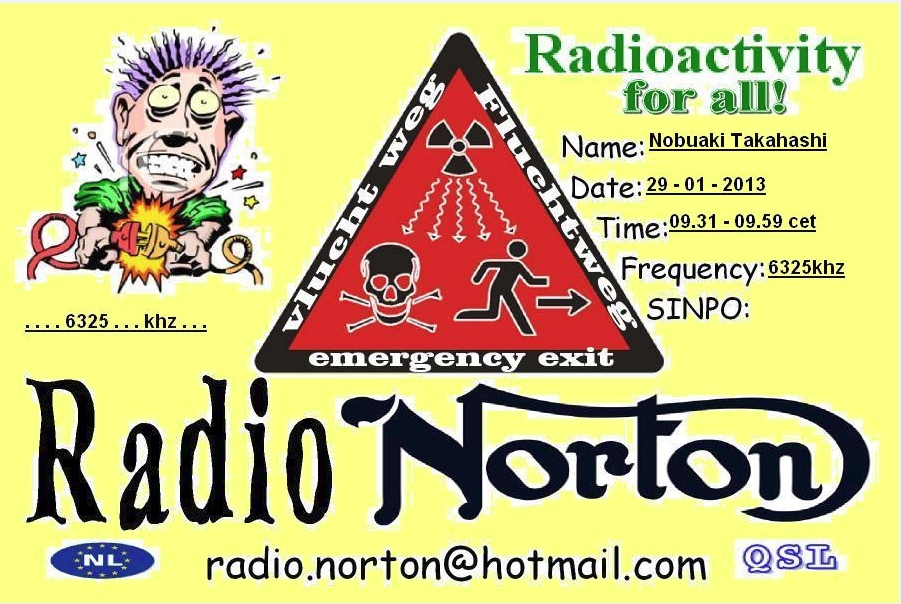The image in question is a digitally created QSL card from Radio Norton, set against a yellow background in a landscape format. Dominating the top left corner, an animated cartoon character, dressed in a green shirt, is depicted being electrocuted while plugging two cords together; his hair stands on end, his eyes bulge, and stars fly around him. Below this, the frequency “6325 kHz” is prominently displayed. 

In the center of the card, a red triangle with black borders houses several warning symbols, including a biohazard icon, a radioactivity symbol, a skull and crossbones, and spiral arrows pointing downwards. Overlaying these symbols is the text "Emergency Exit" along with an image of a silhouette of a person running toward an exit.

In the upper right corner, the phrase "Radio Activity for All" is written in green font. Directly below this are the personal details: "Nobuaki Takahashi, Date: 29-01-2013, Time: 09:31 - 09:59 CET, Frequency: 6325 kHz". The section also includes an empty SINPO field. 

At the bottom, across the center in bold, black font, is the title “Radio Norton,” with the email address "radionorton@hotmail.com" directly beneath it. To the left bottom corner is a logo featuring an oval blue design containing the letters "NL," symbolizing the Netherlands, and at the bottom right corner, the QSL designation is displayed. This QSL card verifies the reception of a broadcast at a specific time and frequency.